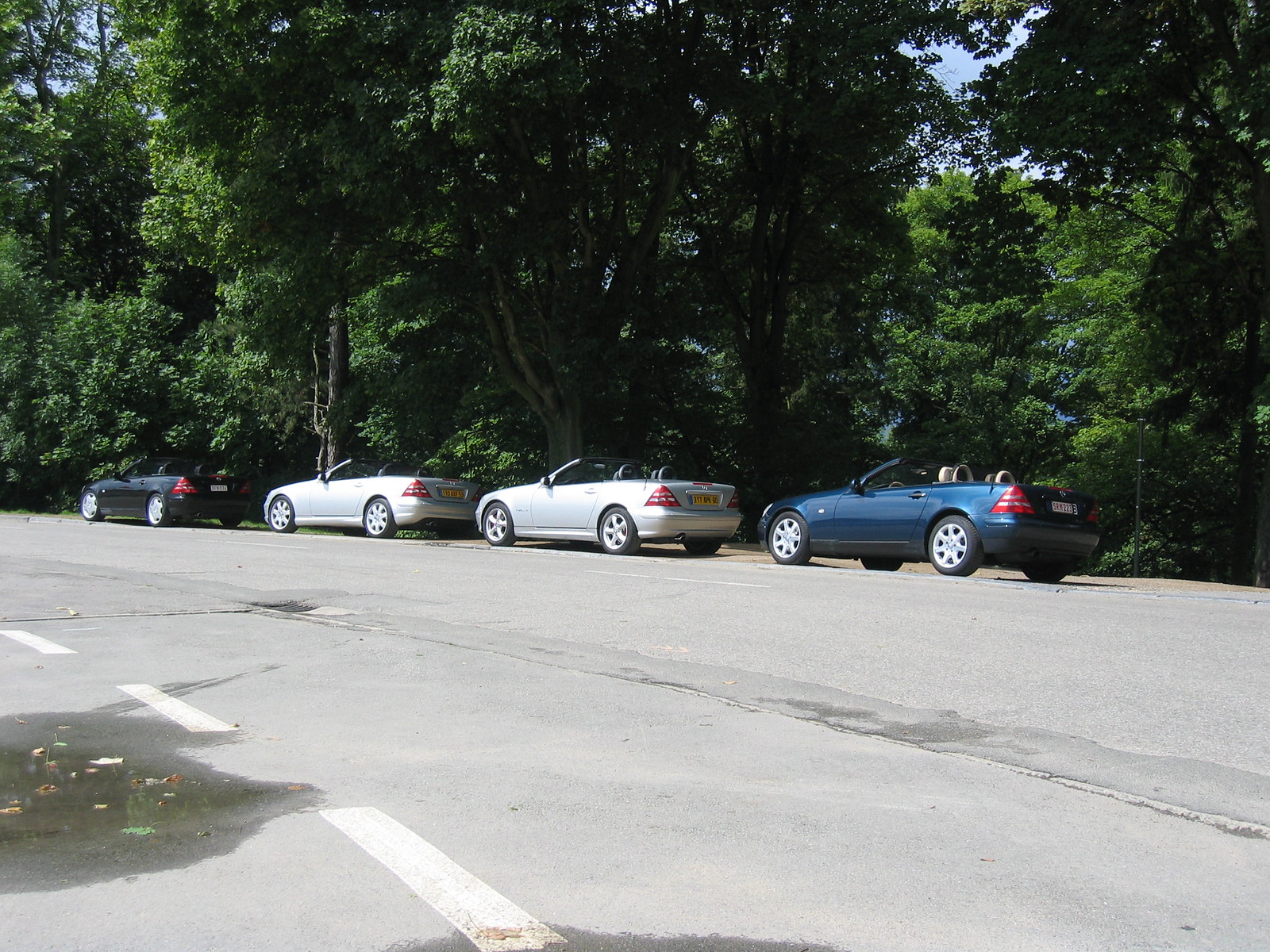This photograph captures a picturesque line of four sleek Mercedes convertibles parked alongside a curved, asphalt highway marked with white stripes. The lineup begins at the right-hand side with a striking black convertible, followed by two nearly identical silver convertibles, and concluding with a deep blue convertible on the far left. All vehicles feature subtle differences in alloy wheels but are otherwise very similar in design, with slanted windshields, red taillights, and visible leather seats. The license plates are of the European style—wider and narrower than typical U.S. plates, suggesting the photo was taken in Europe. In the foreground, subtle details include a cracked road surface and several small puddles, with leaves floating atop the water. The background presents a serene forest of mature, bright green trees, through which glimpses of blue sky can be seen, enhancing the tranquil and elegant setting.